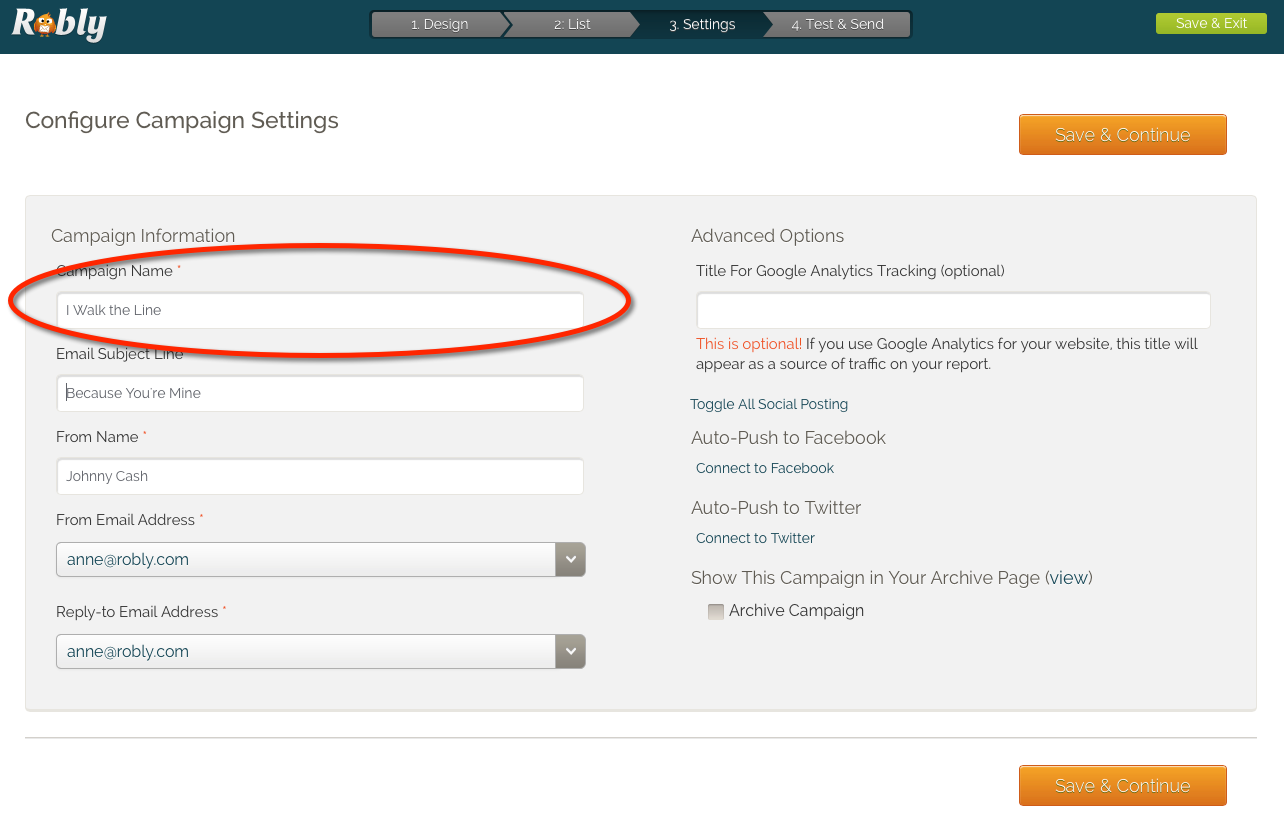The image is a detailed interface of an email marketing platform. At the very top left, there is a label "Robly". Below it, a blue bar divides the sections. On the left side, there is a gray square containing several options labeled as "One Design", "Two Lists", and "Three Settings for Test and Send". Below these, a green button labeled "Save and Exit" is visible. Further down, users can configure campaign settings.

Adjacent to this, there is an orange rectangle labeled "Save and Continue". Another gray square labeled "Campaign Information" is present, with subsections for events, options, and the campaign name. A white bar displays the text "I Walk the Line".

Further details include a prompt for writing a title for Google Net tracking, noting that it is optional but recommended to identify the source of traffic in reports. The email subject line is set to "Because You're Mine". Below that, fields are labeled "From Name" with "Johnny Cash" as a placeholder, "From Email Address" as "name@robly.com," and "Reply To Email Address" also as "name@robly.com".

There are additional text options for toggling social media postings, auto-pushing to Twitter, connecting to Twitter, and archiving the campaign. The interface background is predominantly gray. At the bottom, a horizontal line is followed by another orange rectangle button labeled "Save and Continue".